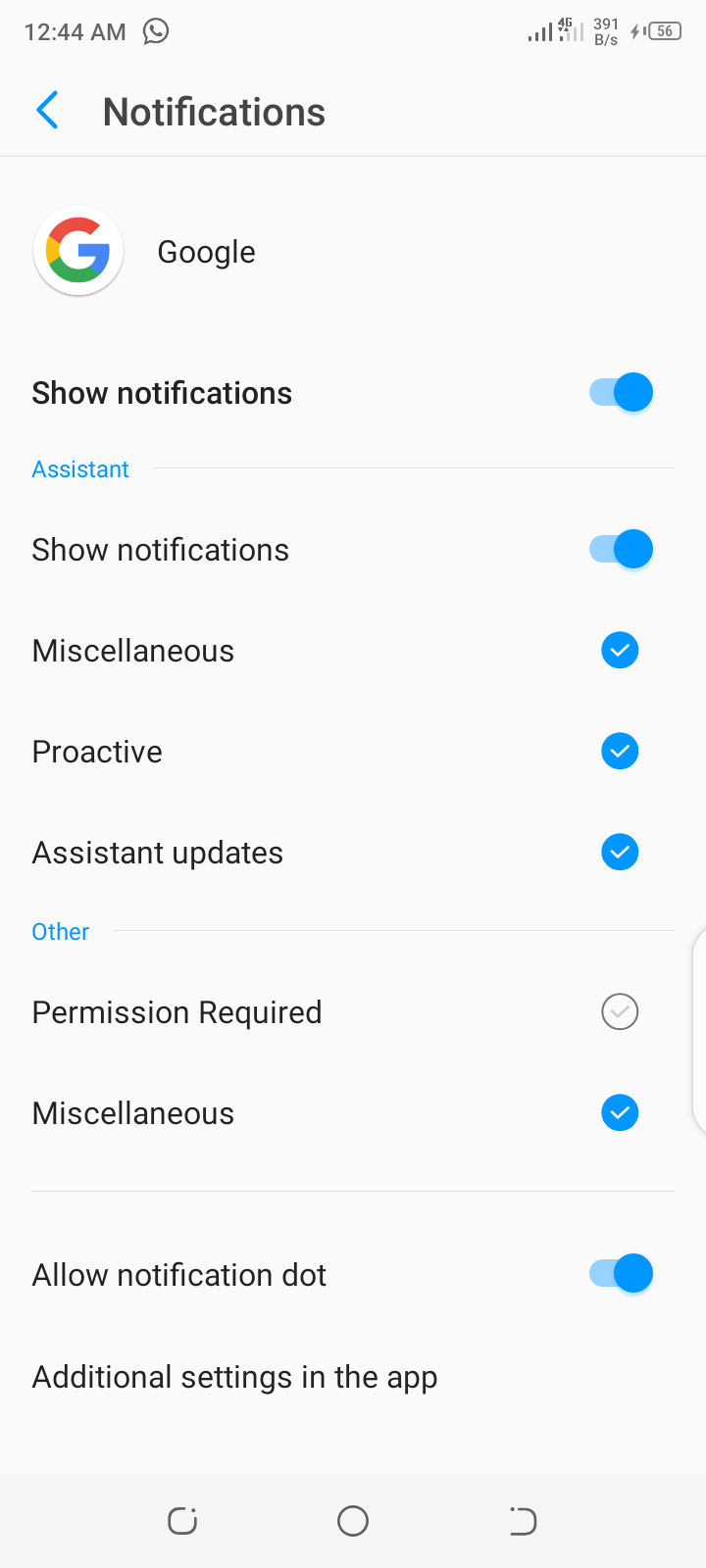Here is a detailed and cleaned-up caption for the image described:

---

**Notifications Menu in the Settings of a Google/Android Device**

At the top left of the menu, there is a blue arrow pointing left, indicating a navigational option to return to the previous menu. To the right of the arrow, in bold gray font, it says "Notifications," separated by a light gray line divider.

Below this header, on a circular white background, there is a Google icon featuring the letter "G" with the top part in red, the left side in yellow, the bottom in green, and the tail in blue. To the right of the icon, in a basic black sans-serif font, it says "Google," followed by the subtitle "Show notifications," which is toggled on.

Another light gray line divider follows, and below it, in small blue text, it says "Assistant." Underneath this, in black font, it states "Show notifications," which is also toggled on, indicated by a red dot in a light blue area to the left.

Further down, in black font, it says "Miscellaneous," accompanied by a filled blue circle with a white check mark to its right. The next section labeled "Proactive" is similarly marked with a filled blue circle and a white check mark. Below "Proactive," it reads "Assistant updates," again with a filled blue circle and a white check mark to its right.

Below another light gray line divider, there is a section labeled "Other" in small blue font. Under the "Other" section, it states "Permission required" in black, with an unselected circular icon outlined in black containing a light gray check mark.

Finally, another "Miscellaneous" section is listed, followed by a filled blue circle with a white check mark, and a segment that reads "Allow notification dot," which is toggled on.

---